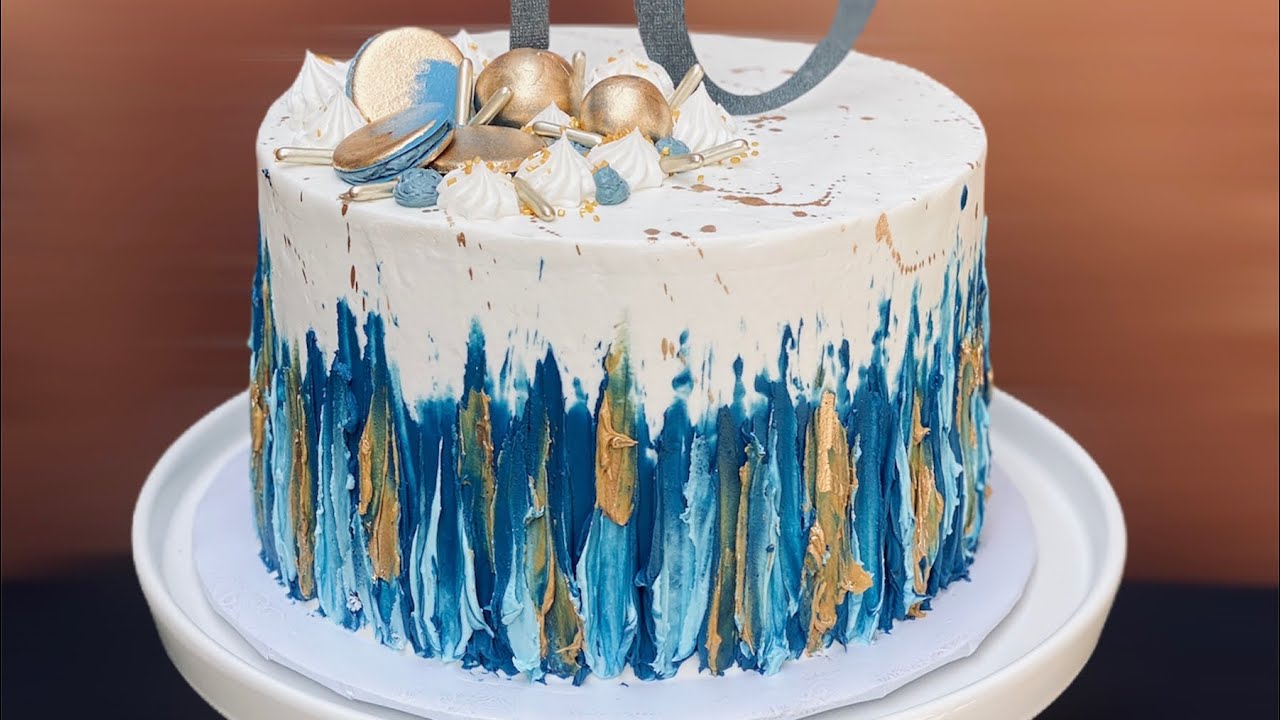The image features a detailed, multi-layered cake set against a backdrop with a rusty, orangish-tan wall and a darker brown surface. The cake is positioned on a white serving tray that itself rests on a white plate with a distinct lip around the edge. The cake, approximately 9 inches in diameter, is predominantly white but showcases a base that combines streaks and points of blue and gold, creating an artistic, upward gradient effect. Adorning the top of the cake are several gold balls resembling Christmas ornaments, gold macaroons with blue filling, blue flowers, and teardrop-shaped white meringue dollops. Additionally, there appears to be a partially visible number on top, though it's cut off and unclear. This elegant cake highlights a blend of intricate decorative elements and striking color contrasts, making it a captivating centerpiece.